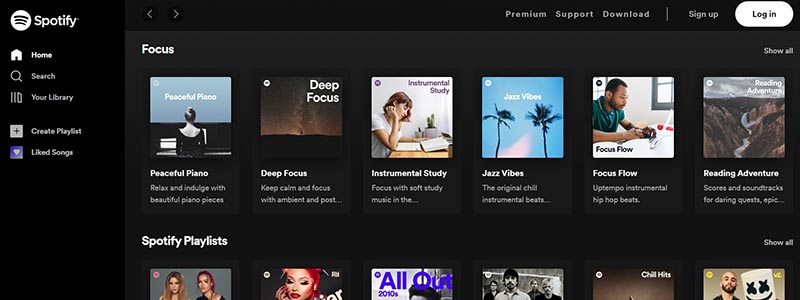This image showcases the Spotify homepage with a sleek black top bar. On the left side of the bar, the white Spotify logo is displayed prominently alongside the word "Spotify." To the right of the logo, there are navigation arrows for backward and forward actions. Further to the right, options for "Premium," "Support," and "Download" are listed, separated by a vertical white line. The far-right corner features the "Sign Up" and "Login" options, with the "Login" button styled in white with black font.

In the main content area, a focus playlist is highlighted. The top right corner includes a "Show All" option in white. The featured playlists are arranged from left to right and include:
1. Peaceful Piano
2. Deep Focus
3. Instrumental Study
4. Jazz Vibes
5. Focus Flow
6. Reading Adventure

Each playlist is represented with a corresponding image and the caption "Spotify Playlist" in white below. There are six more playlists visible below this row, along with another "Show All" button.

On the left side of the page, a vertical menu is displayed on a black background with white font. The menu options include:
- Home (with a home icon)
- Search (with a magnifying glass icon)
- Your Library (with a stack of books or squares icon)
- Create Playlist (with a light gray plus sign)
- Liked Songs (with a blue heart icon)

This detailed layout captures the user interface of Spotify, highlighting its navigation and featured content.